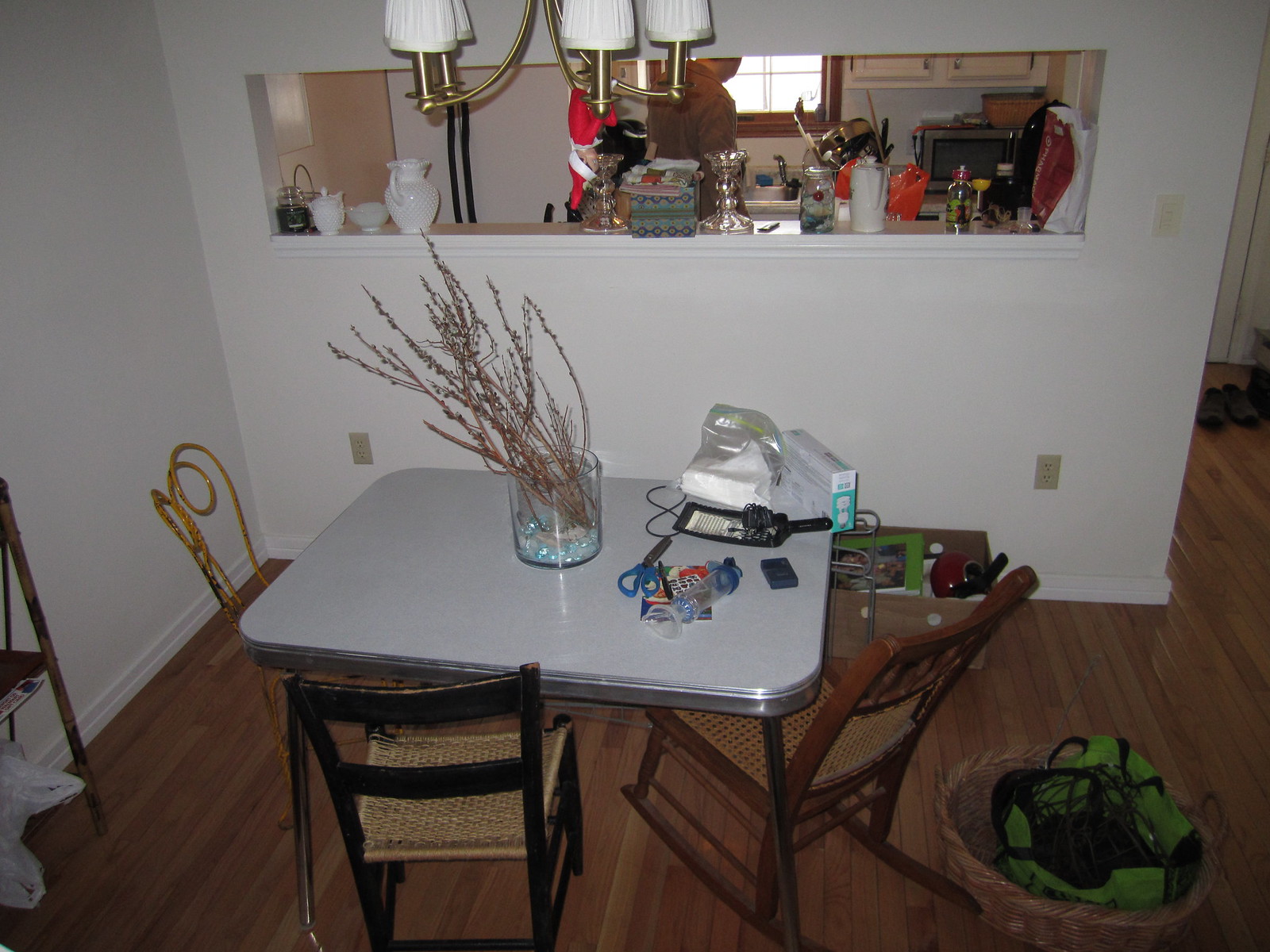The image showcases the interior of a cozy studio or one-bedroom apartment. In the top right corner, the edge of a white door is partially visible, accompanied by a pair of brown shoes placed on the medium brown wooden floor, which features vertical planks running horizontally across the scene. Central to the composition is a square white table with slender silver legs, surrounded by a variety of mismatched chairs including a wooden wicker rocking chair, a black chair with a wicker seat, and a slim chair with a curlicue design on its back.

On the table, there is a plastic container filled with what appears to be wilted plants, contributing to the eclectic clutter. Other assorted items are scattered across the table, adding to the lived-in feel of the space. To the left, a woven basket contains a green helmet. 

A rectangular opening in the wall behind the table offers a glimpse into the adjoining kitchen, where more miscellaneous items are visible. The room contains an array of vases, trophies, and cups displayed throughout the space. Overhead, a gold chandelier with white lantern-style lights adds a touch of elegance to the otherwise eclectic and homey atmosphere.